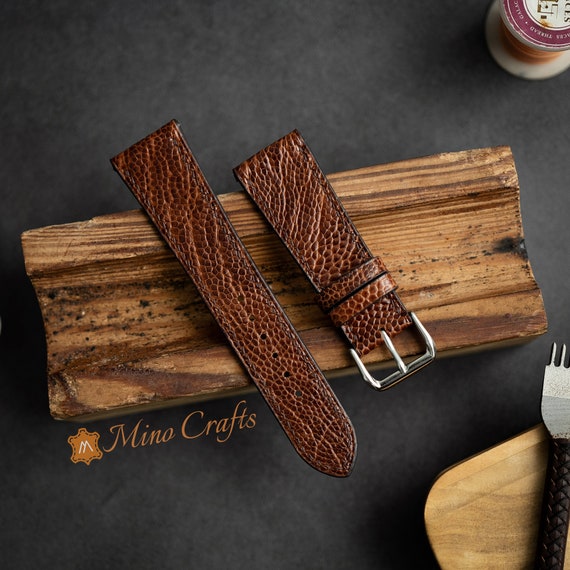The high-resolution image features a beautifully handcrafted brown leather strap with a highly textured, scaly pattern, reminiscent of snakeskin. This strap, which could be part of either a belt or a watch, prominently displays a silver buckle and is artfully posed on a wooden block. Below this central piece, the script "Mino Crafts" is elegantly printed. The backdrop of the image is predominantly black, creating a striking contrast that showcases the detailed craftsmanship of the leather strap. In the bottom right corner, another smaller block of wood holds a black braided leather crafting tool, distinguished by its black braided handle and silver metal tip. The arrangement and high-quality detail suggest the image might be part of an exhibition or sales catalog, emphasizing the luxurious and artisanal nature of the piece.